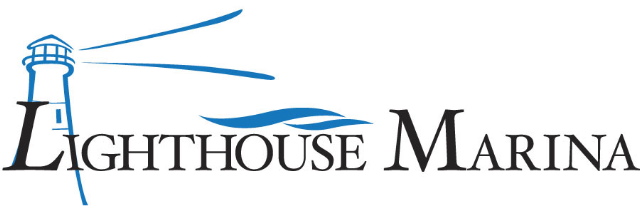The image depicts the logo of a company or place named Lighthouse Marina. The centerpiece of the logo features the words "Lighthouse Marina" in bold black capital letters. Uniquely, the L in "Lighthouse" and the M in "Marina" are significantly larger than the other letters. Attached to the large L is a roughly sketched blue lighthouse outlined in blue but predominantly white inside. This illustration is not fully detailed but includes key features like a roof with a railing and a window. The lighthouse extends downward, intersecting the I in "Lighthouse." Two blue stripes emanate from the lighthouse, suggesting rays of light. Additionally, two blue curved lines positioned above the word “house” in Lighthouse likely represent waves, symbolizing water.